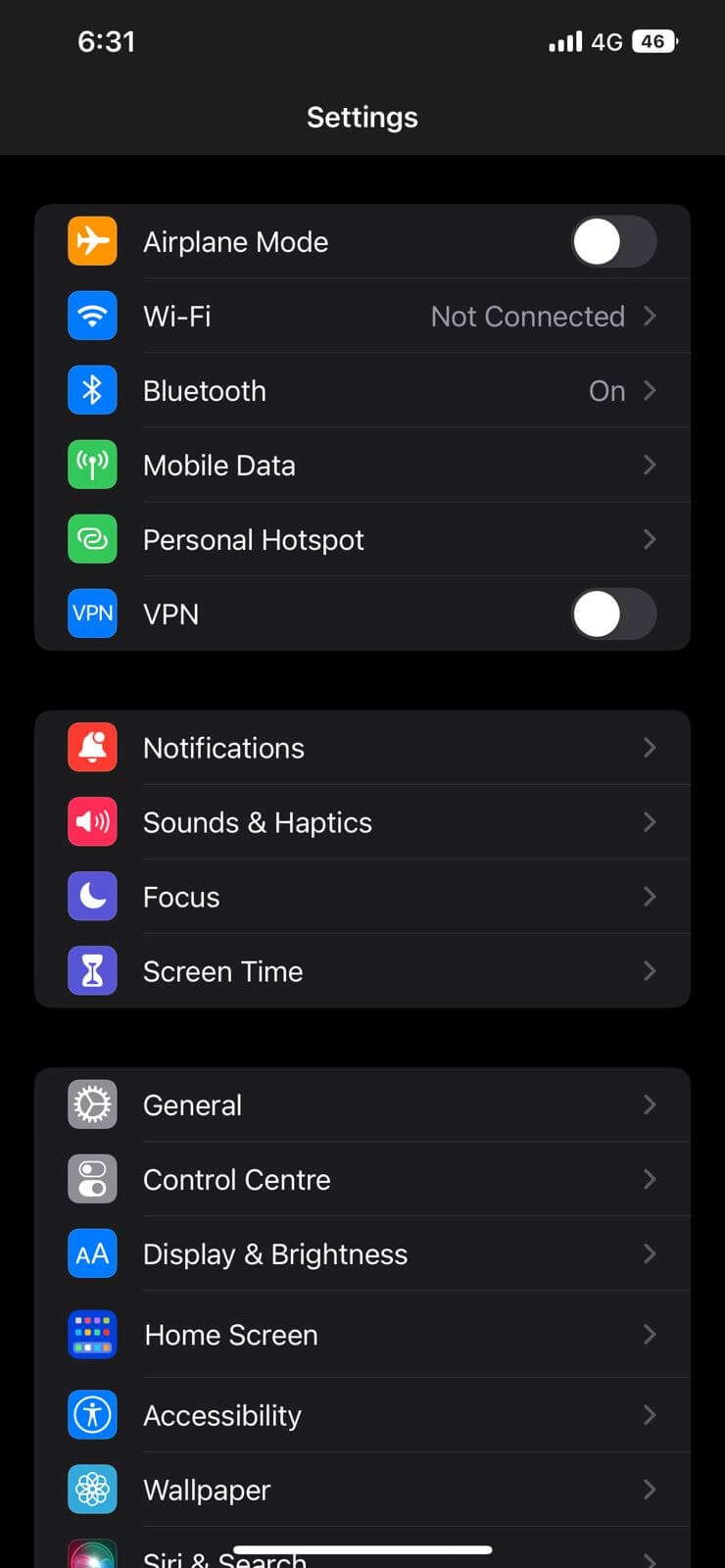The image depicts a settings page on an iPhone, identifiable by the status bar at the top and the distinct "Siri & Search" option. The page features a black header with the word "Settings" written in white. Below the header, a list of typical phone settings is displayed, each accompanied by a colored icon on the left. The settings options include "Airplane Mode" with a toggle switch, followed by "Wi-Fi," "Bluetooth," "Mobile Data," "Personal Hotspot," and "VPN," all featuring similar toggles.

Scrolling further, additional categories such as "Notifications," "Sounds & Haptics," "Focus," and "Screen Time" are present. The subsequent sections encompass "General," "Control Center," "Display & Brightness," "Home Screen," "Accessibility," "Wallpaper," and "Siri & Search." The presence of the "Siri & Search" category confirms that the depicted device is an iPhone. The layout is straightforward, user-friendly, and designed to give quick access to the most commonly used settings, enhancing the overall user experience.